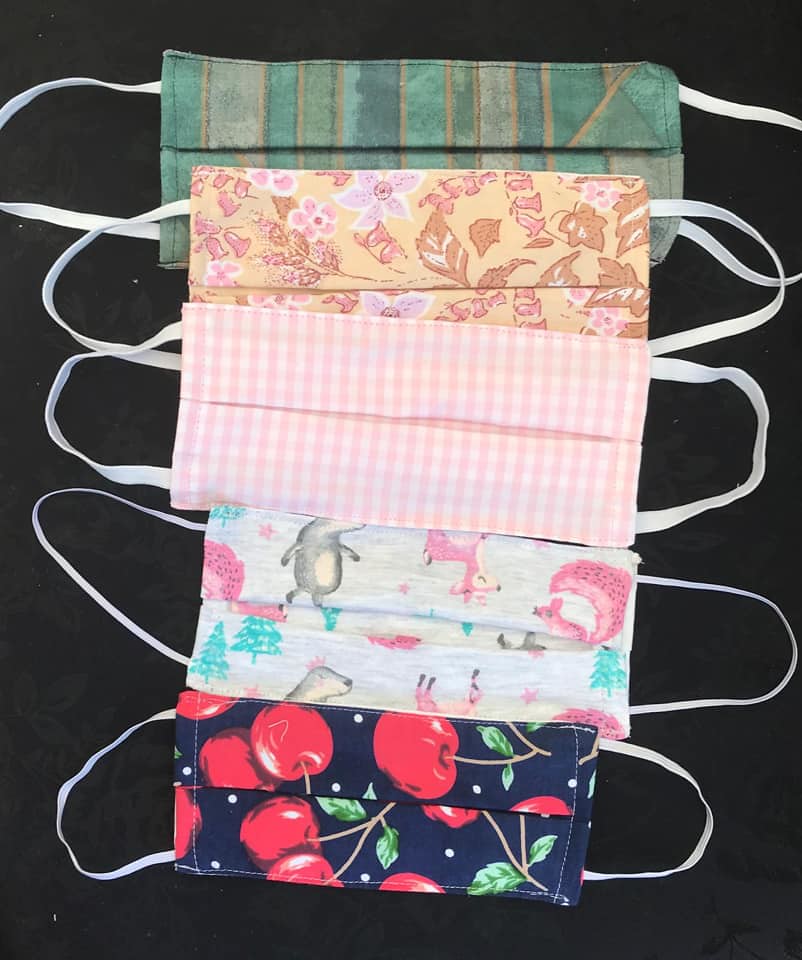In this color photograph with a portrait orientation, five distinct cloth face masks are arranged horizontally against an almost entirely black background, speckled with light brown flecks. Each mask, equipped with white elastic ear loops, showcases a unique design. From top to bottom:

1. A mask featuring an array of vertical stripes in various shades of green, outlined in gold, interspersed with stripes of turquoise.
2. A mask with a beige background adorned with delicate pink and purple flowers, complemented by light brown leaves.
3. A mask displaying a pink and white hatched gingham pattern.
4. A mask with a pale gray or blue background, illustrated with whimsical scenes of pink deer, squirrels, a bear wearing a pink crown, and evergreen trees, all ice skating.
5. A mask with a navy blue backdrop highlighted by large red cherries, bearing brown stalks and green leaves.

Each mask's intricate design, fabric patterns, and contrasting white ear loops make them distinct while fitting within the collective theme of protective yet stylish facial coverings.